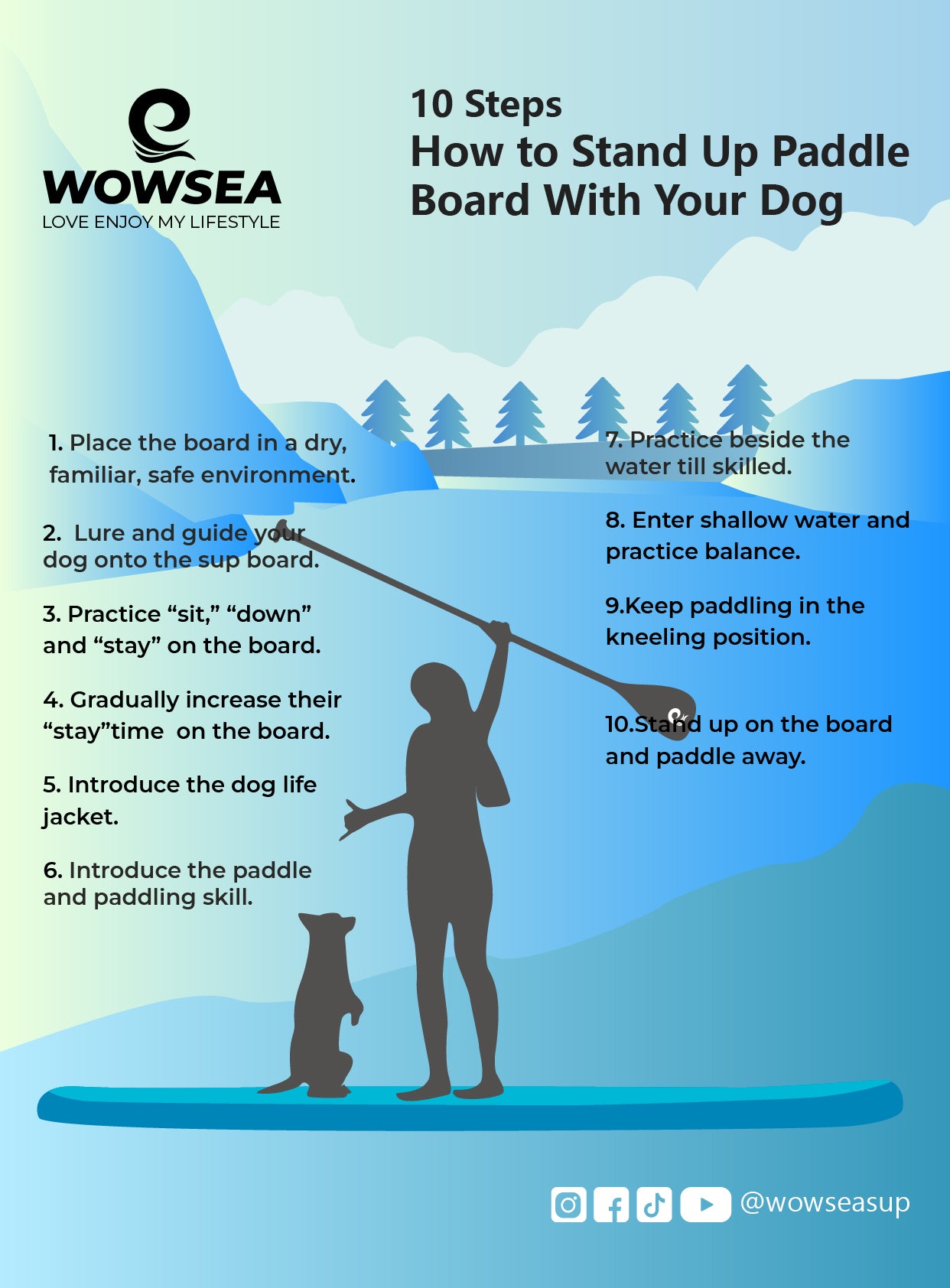This infographic from Wowsee, featuring their logo "Wowsee, Love, Enjoy, My Lifestyle" alongside an ocean wave swirl design, illustrates "10 Steps How to Stand Up Paddle Board with Your Dog." The detailed steps are as follows: 1) Place the board in a dry, familiar, safe environment. 2) Lure and guide your dog onto the SUP board. 3) Practice commands "sit" and "stay" on the board. 4) Gradually increase their stay time on the board. 5) Introduce the dog life jacket. 6) Introduce the paddle and paddling skill. 7) Practice beside the water until skilled. 8) Enter shallow water and practice balance. 9) Keep paddling in the kneeling position. 10) Stand up on the board and paddle away. The image accompanying the steps shows a silhouette of a woman with long hair holding a paddle over her head, standing on a blue paddle board with her dog on its hind legs beside her. The backdrop includes a serene landscape with blue skies, white clouds, mountains, and trees, all reinforcing the tranquil outdoor setting.